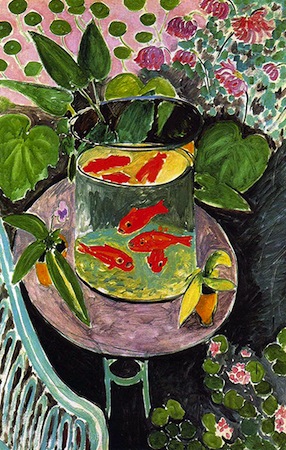The rectangular painting, oriented vertically, features a detailed depiction of a glass cylinder, about three-quarters filled with water, housing four lively goldfish. The base of the cylinder showcases a greenish-yellow substrate, evoking an aquatic environment. This cylinder is elegantly perched upon a pedestal with a distinct purple top, supported by a possibly metallic frame that extends downwards. To the bottom left of the composition, a bench seat subtly makes its presence felt next to the cylinder. In contrast, the bottom right is adorned with a cluster of vibrant flowers, adding a splash of color against the dark, void-like background. The upper section of the painting bursts with life, featuring an array of leaves, petals, and flowers encircling the cylinder, contributing to the lush and natural atmosphere of the scene.